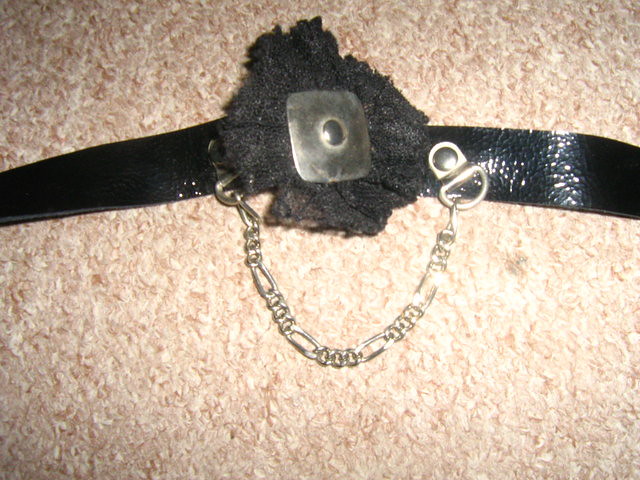The image showcases a black leather strap, approximately a quarter inch thick, laid out on a light brown, textured surface that resembles a carpet or fuzzy blanket. Taken from above with a flash, the strap extends horizontally across the image. At the center of the strap, there is a distinctive ornamental element: a black material designed to replicate the petals of a flower. This flower-like design frames a prominent square, metallic piece with rounded edges, featuring a black circular screw in its center. Flanking this central embellishment is a metal chain with numerous links, running across the front of the strap. The chain has a goldish hue and is securely hooked on each side of the flower-like centerpiece, adding a textured, intricate detail to the overall design of what appears to be a belt or bracelet.